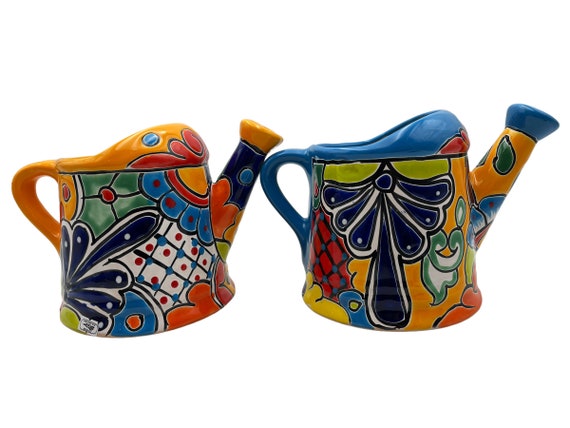This photograph depicts two ceramic teapots set against a white background. Both teapots exhibit vibrant and intricate floral designs, featuring common color themes of blue, orange, green, navy, and yellow. Although their patterns are similar, the color arrangements and specific details differ. The teapot on the left has an orange handle, while the one on the right has a blue handle, with their lids matching these colors respectively. The designs include distinctive blue feathery or petal-like shapes with a striking red and yellow ring at the center, contributing to a funky, cool aesthetic. The handle of each teapot is positioned on the left side, with the spout rising and extending higher than the top of the teapot. The detailed patterns also show a crisscross motif and elements resembling dragonfly wings or structured blue droplets arranged in a semi-circular fashion, with one long droplet descending vertically from the center. These teapots appear to be decorative due to their elaborate designs and atypical material choice for traditional teapots or watering containers.